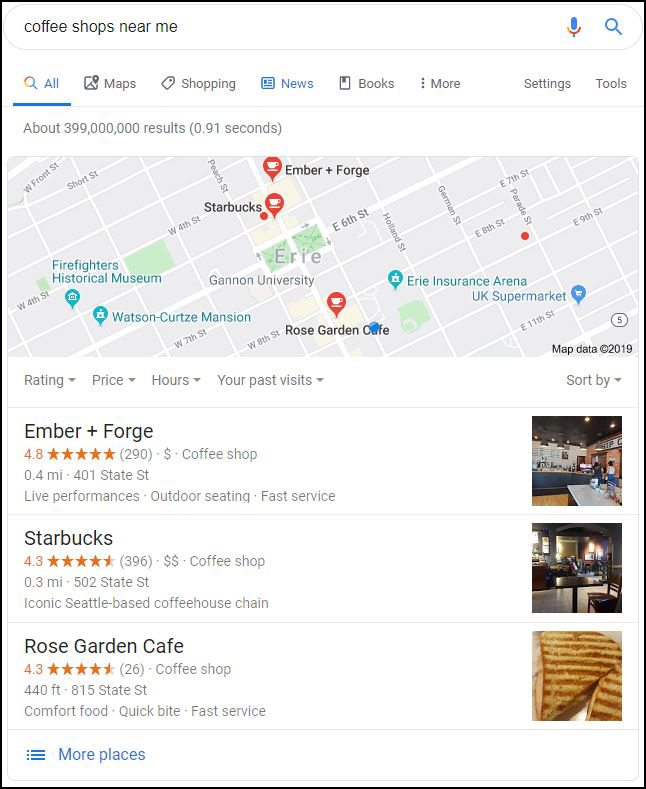This image showcases a user search for coffee shops in Seattle, highlighting three prominent options on a map at the top of the page. The first result is Ember and Forge, boasting a high rating of 4.8 out of 5. This establishment is known for its live performances, outdoor seating, and fast service. The accompanying thumbnail features a long blue counter with various beverages displayed in the background, and a spacious interior with a distinctive black, square-shaped table that can accommodate two to four patrons.

The second result is the iconic Starbucks, renowned as a Seattle-based coffeehouse chain. Its thumbnail displays the typical interior characterized by a blend of brown and beige hues, which is standard across its franchises, ensuring a familiar ambiance whether you're in Seattle, Chicago, New York, or elsewhere.

The third and final result is the Rose Garden Cafe, which shares a 4.3 rating with Starbucks. It offers comfort food, quick bites, and speedy service. The thumbnail shows a brown cookie flecked with chocolate, resembling a striped graham cracker. This cafe is located a bit farther at 815, but all three coffee shops are conveniently situated close to one another on the same block, making it easy for the user to find a decent coffee spot in this neighborhood.